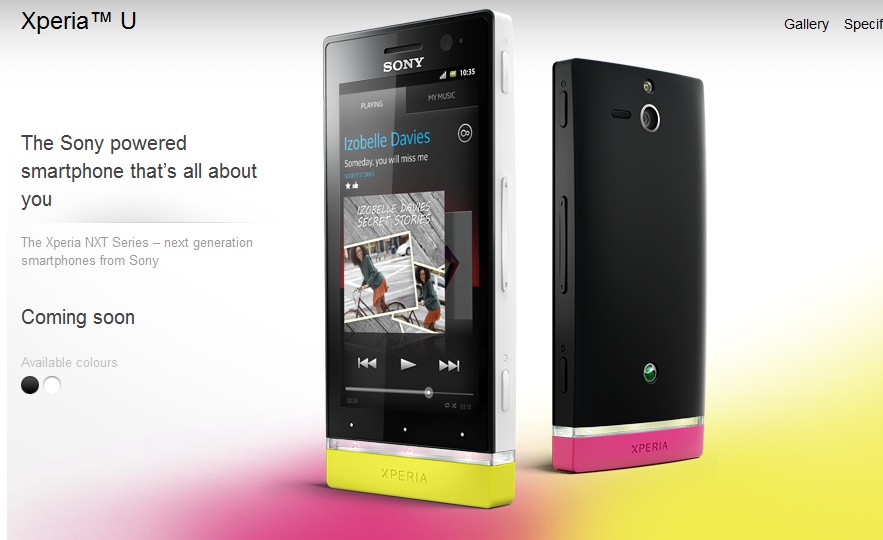This advertisement for the Sony Xperia U is a detailed showcase of the smartphone. In the top left corner, the text displays "Xperia™ U" followed by the tagline "the Sony-powered smartphone that's all about U." Beneath that, in smaller text, it states: "The Xperia NXT series, next generation smartphones from Sony." Further down, in the same prominent font, it reads "Coming soon," and in smaller print, "available colours: black and white."

The advertisement features two versions of the Xperia U phone. On the left is a front view of a black phone with a yellow bottom part, which prominently displays "Xperia" on the lower section of the screen. The screen shows it's playing a song by Isabel Davies titled "Someday You Will Miss Me." To the right, slightly behind, there is a back view of another phone with a black top and pink bottom part, revealing the camera positioned at the top.

The background of the ad transitions from gray at the top, fading to white and then changing to yellow on the lower right and pink at the bottom center. In the upper-right corner, partially cut off, is the black print text "Gallery S-P-E-C-I-F..."

Overall, the image effectively highlights the Sony Xperia U’s unique design features, available colors, and upcoming release.